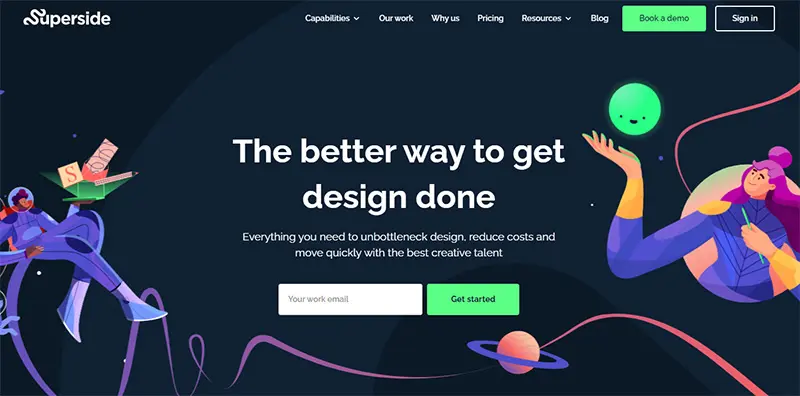This image features a promotional design for the website Superside, set against a sleek black background. In the top left corner, the Superside logo is prominently displayed. The top navigation bar, extending across the page, includes links labeled Capabilities, Our Work, Why Us, Pricing, Resources, and Blog. To the right, two buttons are displayed: a vibrant green button labeled "Book a Demo" and a dark button labeled "Sign In."

Dominating the center of the page, bold white text reads "The Better Way to Get Design Done." Beneath this, in smaller, supportive text, it elaborates: "Everything You Need to Unbottleneck Design, Reduce Costs, and Move Quickly with the Best Creative Talent." Below this text, a subscription box prompts users to enter "Your Work Email" alongside a green button with black text inviting them to "Get Started."

A captivating, large-scale illustration spans the width of the page. On the far left, a stylized figure in a purplish-blue spacesuit stands against a cosmic backdrop, cradling an intriguing box emitting an "S," a pencil, and an envelope with a card. On the far right, another figure—a woman with striking purple hair—wields a pencil in her left hand while her right hand reaches toward a whimsical green planet with expressive eyes and an open mouth hovering just above it. At the very bottom of the page, a celestial body adorned with a blue or purplish ring completes the space-themed artistry.